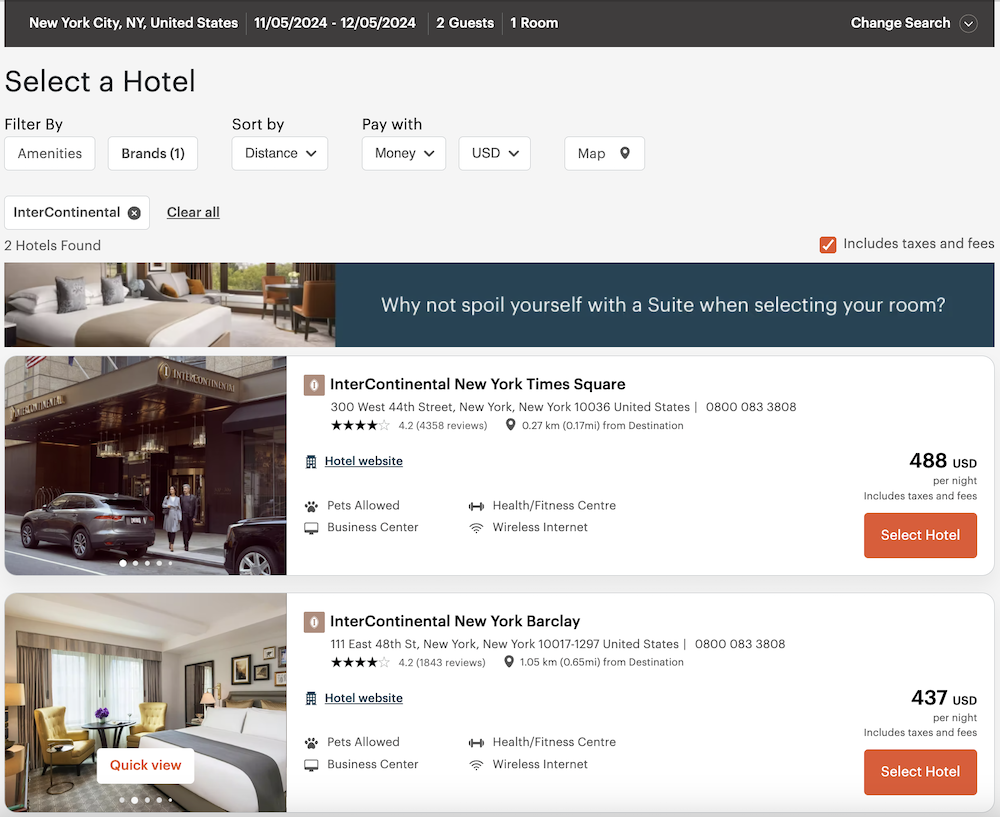This image captures a screenshot of a travel website interface. At the top, a header in black and white text states, "New York City, New York, United States," followed by the dates "11/5/2024 through 12/5/2024." It also specifies "Two guests, one room." In the upper right corner, there is a "Change Search" option with a pull-down menu button. The interface below this section features a gray background with filters and options for refining the search, including "Select a Hotel," "Filter by Amenities," "Brands," "Sort by Distance," "Pay with Money" (also featuring a pull-down menu), and options for currency ("USD") and viewing a map.

Beneath these controls, the results display images of two hotels matching the search criteria. The first result is "Intercontinental New York Times Square." To the left of this text, there's a color image of the hotel entrance on a bustling city street, featuring two people walking in front of the entrance.